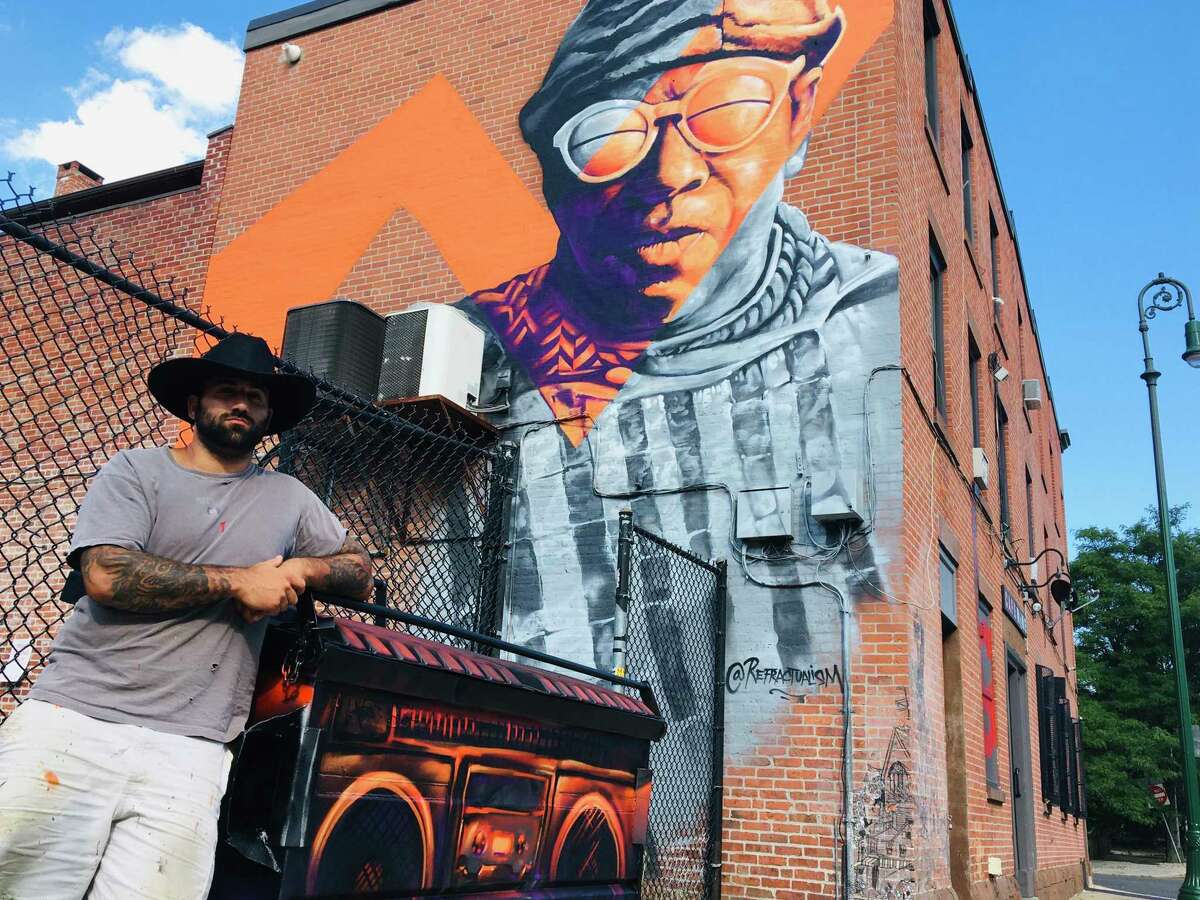In this brightly lit outdoor scene, a man with tattooed forearms stands against a chain-link fence, leaning on a trash can painted to resemble a stereo. He sports a black cowboy hat, black beard, a gray t-shirt, and dirty white pants. Positioned on the left side of the photograph, the viewpoint looks slightly upward towards him. Behind the man, a three-story brick building displays a striking mural of an African-American figure in a military-style outfit, wearing sunglasses with horizontal slits and featuring only the face in color. An artist’s signature, "refracturalism," is visible at the bottom of the mural. The mural is accented by a thick, orange zigzag line running through it. In the background, a blue sky with a few clouds, a green streetlight, a "Do Not Enter" sign, and some trees are visible, adding depth to the urban scene.